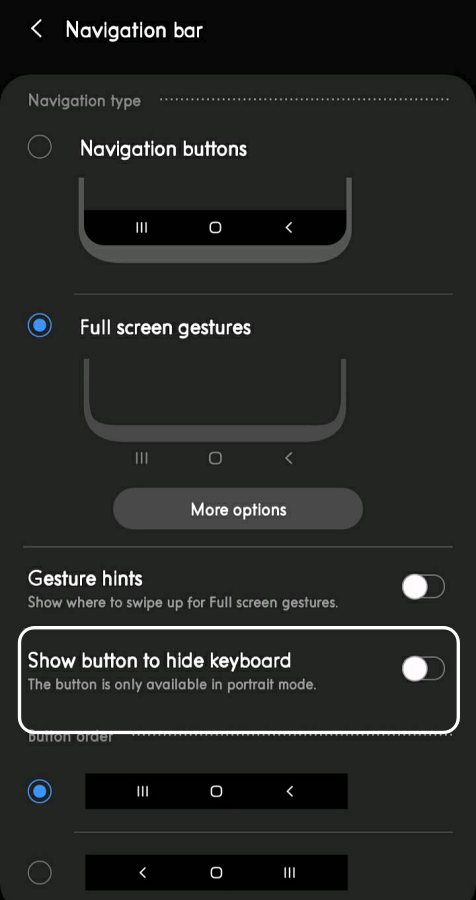This image showcases a detailed mock-up of a website's navigation bar. At the very top, the text "Navigation Bar" is displayed in white on a black background, with a left-facing arrow adjacent to it. Directly beneath, "Navigation Type" is written in dark gray text.

Below "Navigation Type," a circular icon is labeled "Navigation Buttons." The illustration includes the bottom segment of a phone with rounded edges. On this phone’s bottom section, there are three distinct icons: three horizontal white lines on the left, a white circle in the middle, and a left-facing arrow on the right.

Further down, the caption "Full Screen Gestures" is displayed in white text. To the left of this caption is a circle, consisting of a white outlined outer circle and a solid blue inner circle. The mock-up reiterates the phone’s bottom section.

Next, a rounded gray rectangle containing the white text "More Options" is visible. Below this is a horizontal white line followed by the text: "Gesture hints: show where to swipe up for full screen gestures" in white. To the right of this text is another circle containing a left-facing arrow.

Further down, an outlined white box states, "Show button to hide keyboard. The button is only available in portrait mode." Another white circle accompanies this text.

At the very bottom, the text "Button Order" is presented, accompanied by a white circle with a solid blue inner circle. Additionally, the imagery of the three white lines, the white circle, and the left-facing arrow reappears.